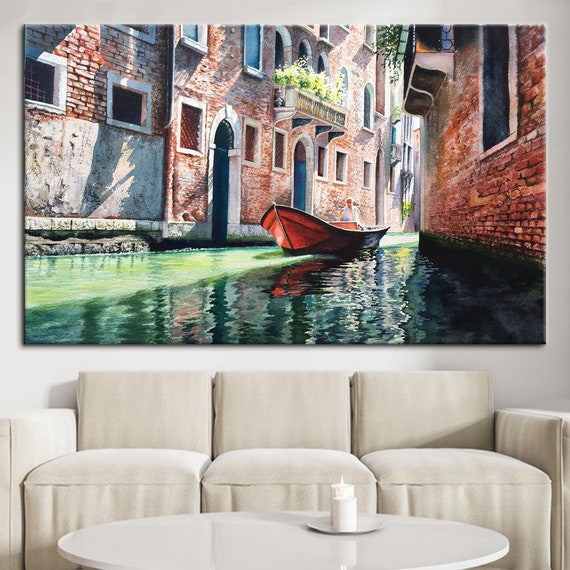The image showcases a sophisticated front room or seating area. Dominating the scene is a plush three-seater couch upholstered in a pale beige velour material, featuring straight arms and a straight back. Positioned directly in front of the couch is a sleek, oval-shaped white table accented with a high-shine finish. On the table's right side, two pure white candles rest atop a white china plate, with the candle furthest from the camera gently flickering.

The focal point of the room is a high-quality, frameless painting mounted on the white wall above the sofa. This exquisite artwork depicts a serene riverscape reminiscent of a Venetian canal. The greenish river, shadowed and illuminated by the sun's interplay with the surrounding buildings, flows between red brick houses adorned with arch-shaped doorways framed in marble. Some balconies are decorated with plants. A wooden boat, its bow raised, gently cruises down the river, with a lone figure clad in white standing aboard. The painting masterfully captures the reflections of both the boat and the buildings in the murky, greenish waters, adding depth and realism to the scene.